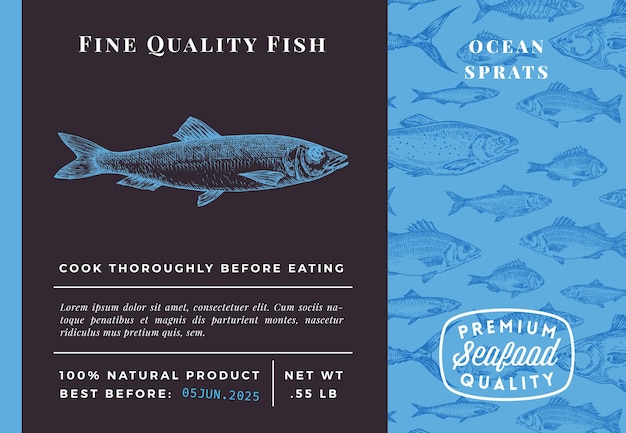This image is a detailed food label or sales poster for a seafood product named "Ocean Sprats." The design is divided with the left two-thirds of the poster in black and the right one-third in blue.

In the black section on the left, there are white text elements prominently stating "Fine Quality Fish" at the top, followed by a blue line drawing or x-ray image of a fish. Beneath this image, in smaller white text, are the instructions "Cook Thoroughly Before Eating" followed by other text that appears less clearly but includes, "100% Natural Product," "Best Before 05 JUN 2025," and "Net Weight 0.55 lb."

The right blue portion of the image is patterned with darker blue outlines of various fish swimming in different directions. This area features the product name "Ocean Sprats" in white text and at the bottom, the phrase "Premium Seafood Quality."

Overall, the design emphasizes the high quality and natural attributes of the product, providing necessary consumer information clearly and attractively.